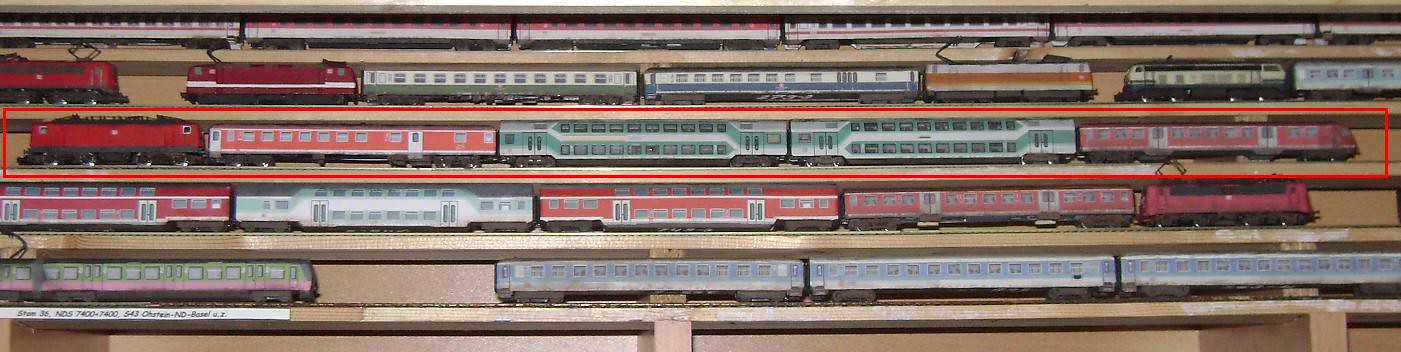This image is a highly horizontal and detailed depiction of multiple model train cars displayed on wooden shelves, arranged in at least five or six rows. The trains appear to be modeled after old-timey boxcars with numerous windows. In the center of the image, a red rectangle is prominently outlining a specific train set in the third row, which includes a red and black engine followed by a series of cars. These cars are colored in various shades: two are turquoise green with white windows, another is entirely red, and one is orange and white striped. The trains throughout the shelves display a diverse palette, featuring colors such as dark grey, white, green, blue, and orange. At the bottom left of the display, a small white piece of paper stuck to the shelf likely denotes the names or details of the train sets. The area between the shelves and trains has a shiny gold appearance, adding a touch of elegance to the otherwise dense and intricate arrangement.